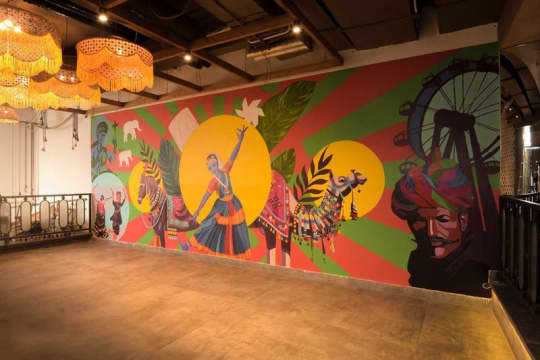The photograph features a large, open space with high ceilings accented by wooden framing and illuminated by lights at the joints. Several tassel-adorned lanterns hang from the ceiling, casting a warm glow on the scene below. The focal point of the room is a grand mural that covers an entire wall, depicting a vibrant and dynamic scene suggestive of Indian or Middle Eastern art influences.

In the center of the mural, a woman dressed in a traditional teal blue and orange costume strikes a dramatic pose, with one arm raised expressively and the other lowered toward the ground. She stands against a backdrop of symmetrical yellow circles, green and pink radial lines, and a large yellow sun behind her. To her right, a camel adorned with a pink cloth and decorative beads is depicted. Its detailed harness, rings, and pom-poms add to the ornate look.

On the left side of the mural, two women in traditional outfits engage in a dance. One is dressed in a brown tunic and knee-length skirt, while the other wears a full-length outfit with a pale red top and dark brown skirt. The mural also features a horse with a cocoa-brown coat, decorated with floral garlands and other ornamental designs, alongside a male figure wearing a turban, positioned near a Ferris wheel suggesting a festive or circus atmosphere. Intricate elements such as small white elephants and religious symbols are interspersed throughout the mural, adding to the complexity and richness of the scene.

The floor below the mural resembles tan-colored tile, possibly a dance floor, with decorative iron railings on either side of the space. An iron-gated area to the left hints at a dining or gathering space beyond. The room is impeccably prepared, seemingly waiting for a performance or event to unfold.